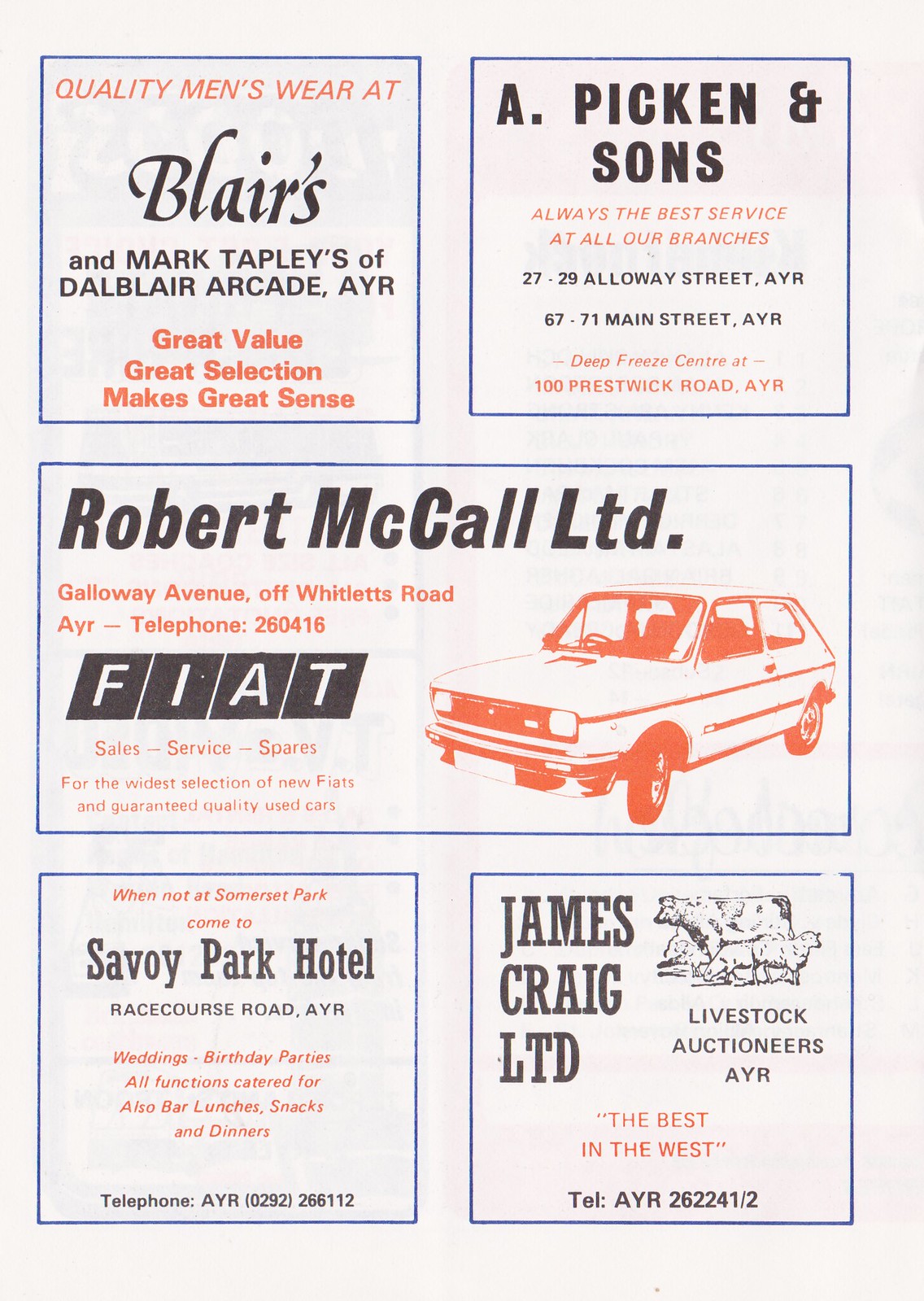The image is of a retro advertisement page on an off-white paper with a blue border, likely from a magazine or newspaper. The page features five distinct advertisements, each in its own box with a combination of red and black text.

In the top left box, there is an ad for Blair's featuring the phrase "Quality Menswear at Blairs" in red on a white background, with "Blairs" in black. Below, it lists the address "Taples of Dale Blair Arcade, AYR." At the bottom, in red text, it proclaims, "Great Value, Great Selection, Makes Great Sense."

To the right, the top right box advertises "A. Pickens and Sons," using alternating black and pink fonts to state "Always the Best Service at All Our Branches," followed by addresses: "2729 All the Way Street, AYR," "671 Main Street, AYR," and "100 Prestwick Road, AYR."

The center of the page has a large, full-width ad for "Robert McCall Limited" with bold black letters on a white background. Directly beneath, in white letters on a black background, it declares "Fiat," with a drawing of a Fiat car depicted in red on the white background.

In the bottom left box, an ad for "Savoy Park Hotel" presents the message: "When Not at Somerset Park, Come to Savoy Park Hotel" in small red print, followed by the address "Racecourse Road, AYR" in black.

Finally, the bottom right box promotes "James Craig Limited," featuring a drawing of a cow and the tagline "Livestock Auctioneers" in black. In red text, it asserts "The Best in the West," with a phone number listed below in black.

The entire layout combines a nostalgic design with a straightforward color scheme of black and red, encapsulating the charm of vintage advertising.